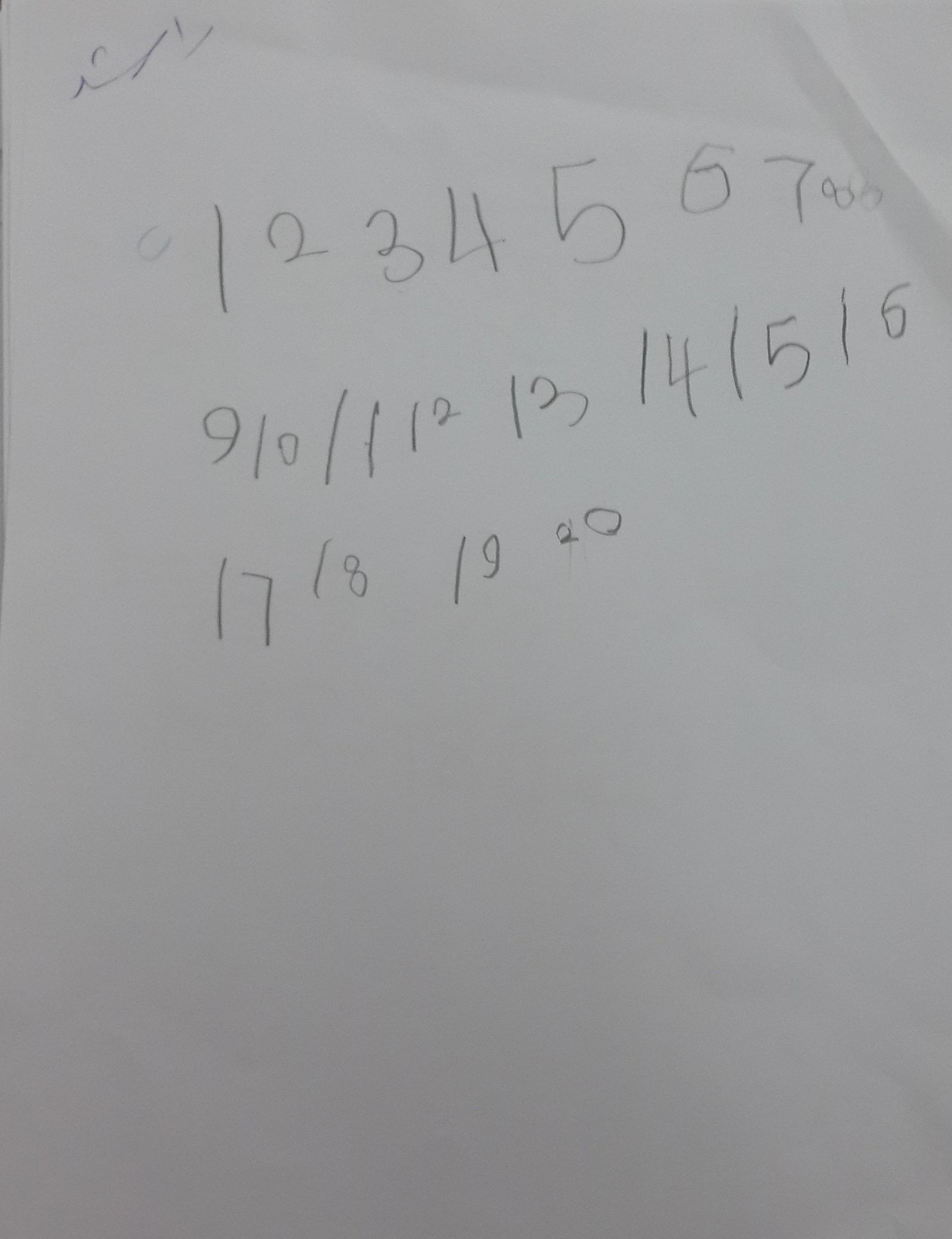The image showcases a full shot of a piece of paper, likely pale grey but possibly white under poor lighting. The paper features various numbers hastily scribbled in pencil. In the top left corner, there are additional indistinct pencil scribbles. The top right corner of the paper is noticeably creased, indicating it has been bent. The numerals are arranged in a somewhat haphazard manner:

- The first row contains the sequence: 1, 2, 3, 4, 5, 6, 7, followed by two instances of the number 8.
- The second row presents the numbers: 9, 10, 11, 12, 13, 14, 15, and 16.
- The third row lists: 17, 18, 19, and 20, with the number 20 showing a correction where 1 has been partially erased and overwritten by 2.

The numbers are written without any commas separating them and exhibit a lack of uniformity, suggesting they might be the work of a child practicing their handwriting.